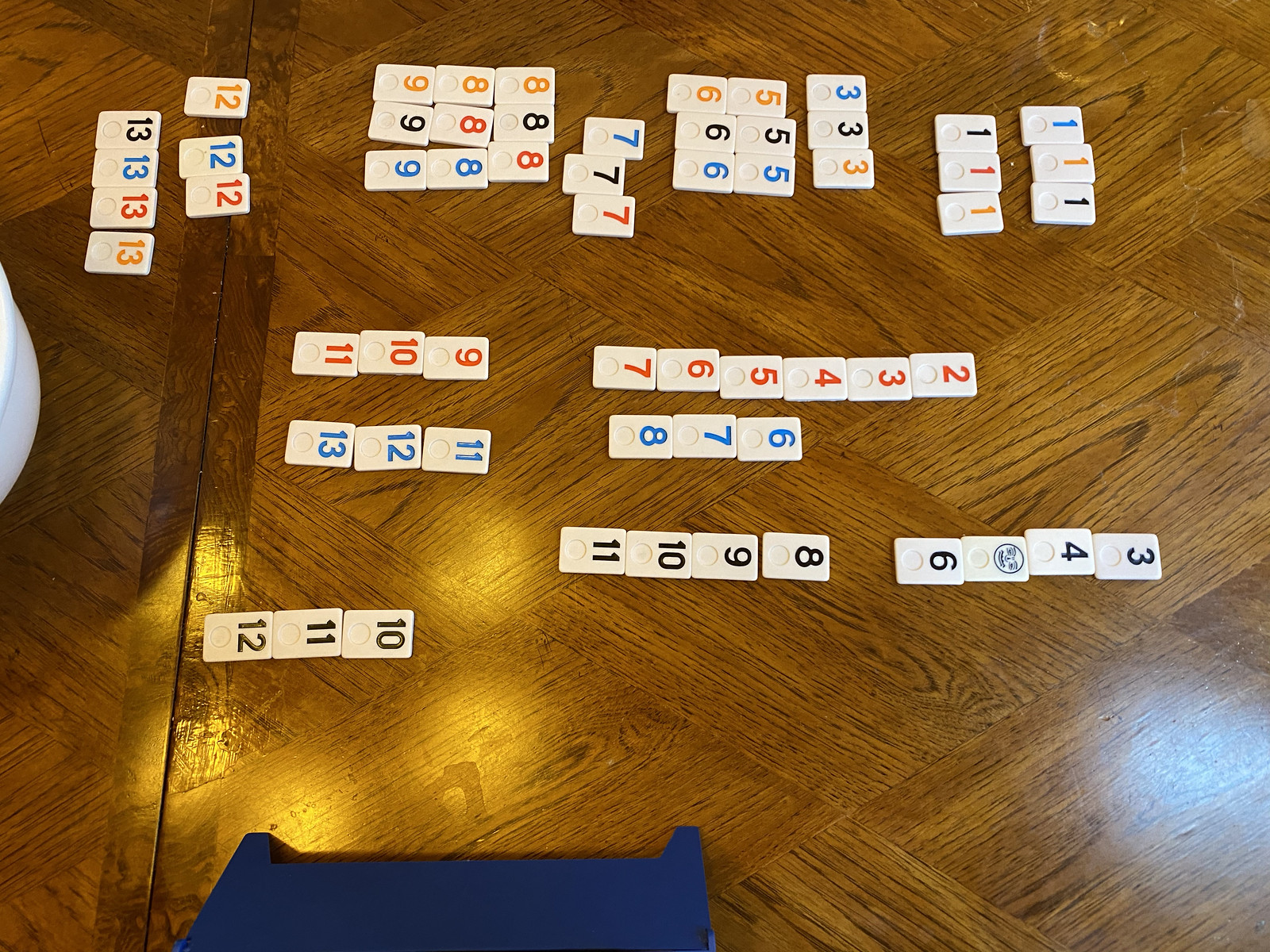This image shows a meticulously arranged set of around 30 dominoes on an elegant wooden floor. The floor itself boasts a distinctive diagonal, almost checkered pattern created by alternating wood grain directions, adding a rich visual texture to the scene. The dominoes, some in clustered groups of three, four, or five, are spread across the frame with a few notable formations. On the left, we glimpse what appears to be a person's knee, hinting at someone in the act of setting up the arrangement, cropped out just slightly from the edge of the photo. Towards the bottom, there's a sequence of four dominoes clearly numbered 13, lying in a neat row. Adjacent to this, a vertical column stacks numbers 10, 11, and 12 in descending order. The colorful assortment of the dominoes—coming in black, blue, red, yellow, and possibly orange—contrasts against the warm hues of the wooden floor, creating an engaging and visually intriguing composition.